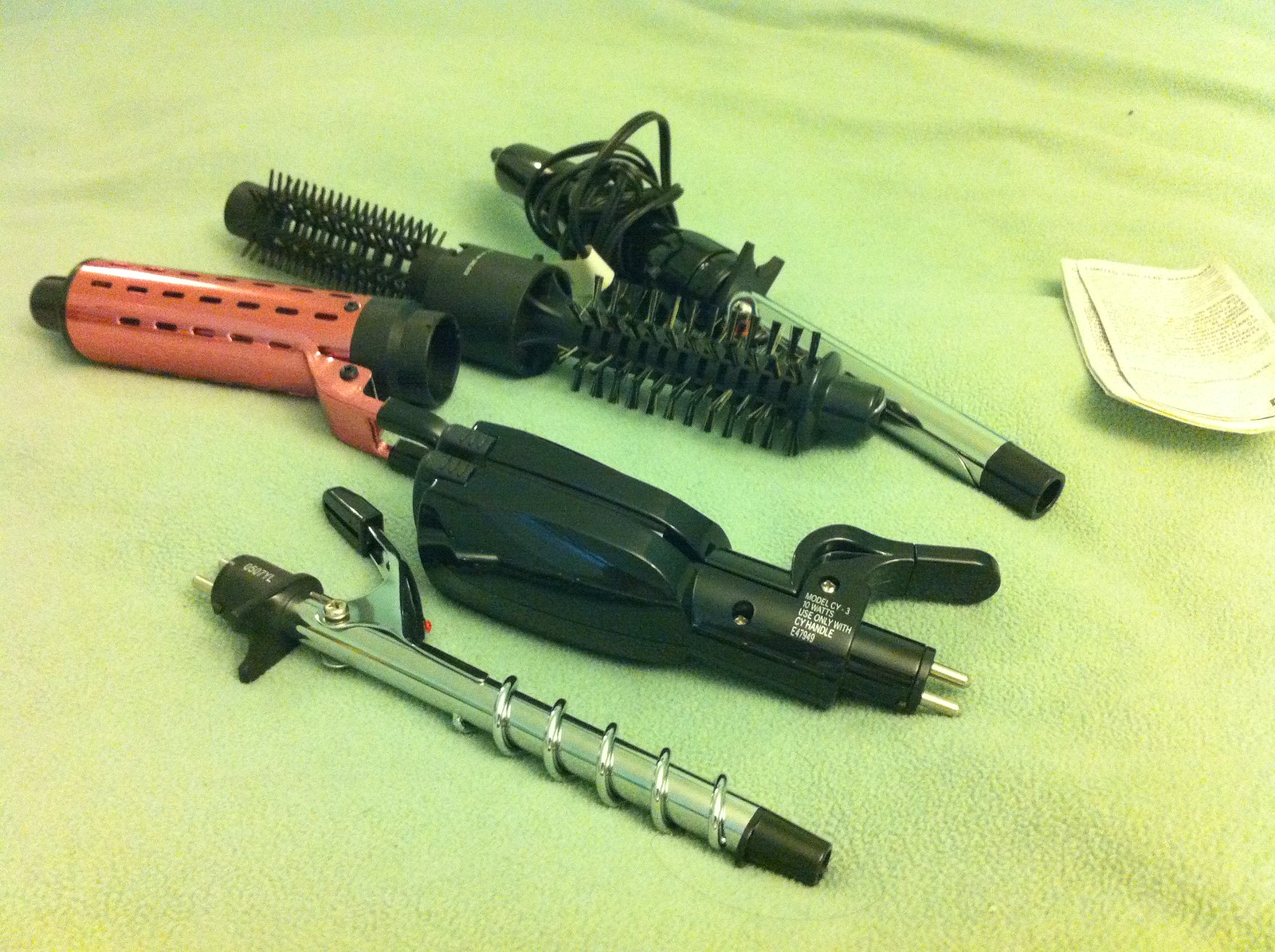This detailed photograph showcases an array of grooming tools meticulously arranged on a lime green to yellow blanket. In the backdrop, a standard curling iron with its black handle wrapped in a cord and a chrome blade stands out. Adjacent to it is a cylindrical brush attachment, designed for use with other hair equipment. Below, a comb attachment and an orange attachment with a larger round head are positioned side by side. Accompanying these is a potential clipper attachment. In the forefront, a distinctive spiral curling iron attachment, featuring a spiral chrome design for wrapping hair, completes the collection. The black hair straighteners with silver metal tips add a sleek touch to the assortment, highlighting the variety of tools meant for hair styling and grooming.